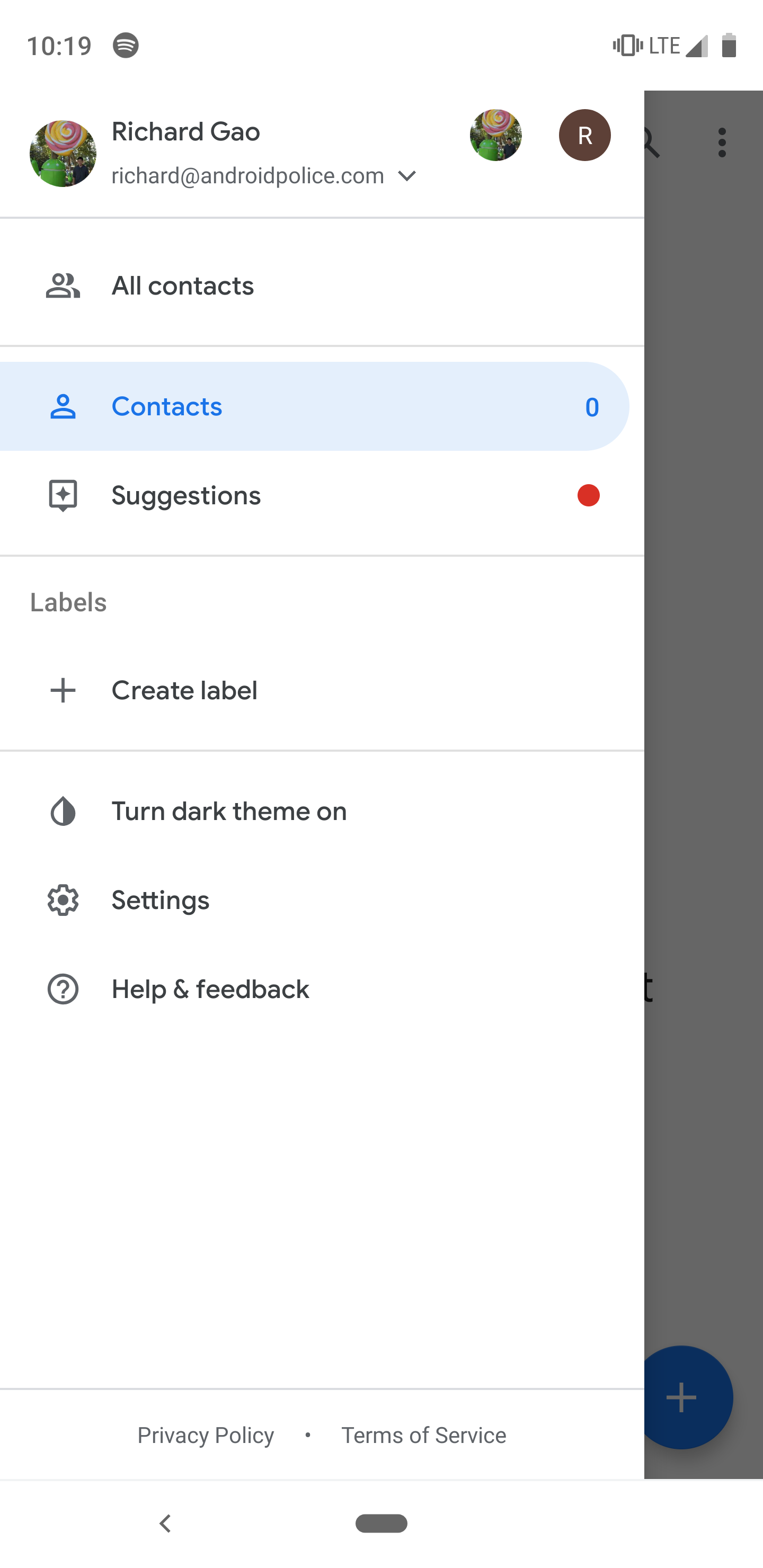This vertical screenshot captured from a smartphone device predominantly features a white background, likely from a computer screen with a pale gray vertical strip running along the right-hand side. In the top left corner, the current time is displayed as 10:19, accompanied by a small icon. Moving to the right, additional icons can be seen, including a mostly filled LTE signal strength icon and a battery life indicator.

Towards the left side, a small circular profile picture labeled "Richard Gao" is displayed along with his email, "Richard at androidpolice.com". Next to this is another circular icon, brown with a white "R" on it. 

Below this section, navigation options are visibly separated by lines. The first labeled section reads "All contacts", followed by another icon labeled "Contacts", highlighted in blue with a zero beside it. Underneath is a "Suggestions" category marked with a filled red circle on the right. Following another dividing line, there's the "Labels" section accompanied by a plus sign indicating "Create label". Further down, an option to "Turn dark theme on" appears, followed by "Settings", and lastly, an icon with a question mark labeled "Help and feedback".

At the bottom of the screen, separated by another line, "Privacy Policy" and "Terms of Service" are displayed with an arrow pointing to the left directly under the terms of service text, indicating navigation or a back option, ending with a thicker line underneath.